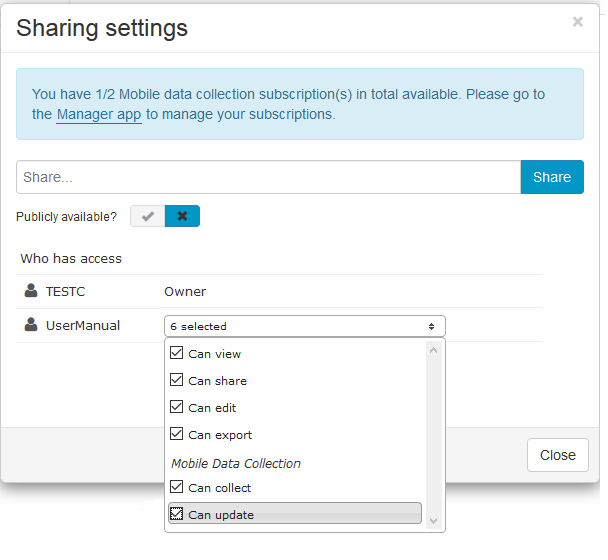Screenshot Description: Settings Screen

The image depicts a settings screen with a clean, minimalist design on a white background. 

**Top Section:**
- *Upper Left Corner:* In bold black font, the heading "Sharing Settings."
- *Upper Right Corner:* A gray "X" icon for closing the screen.

**Central Area:**
- *Notification Box:* 
    - Background: Light blue with a border.
    - Text: "You have half mobile data collection subscriptions in total available. Please go to the manager app to manage your subscriptions."

**Interactive Elements:**
- *Drop-down Menu:* 
    - Label: "Share"
    - Button: Blue with white text, labeled "Share."
- *Publicity Status:* 
    - Text: "Publicly Available"
    - Indicators: A checkmark (not pressed) and an "X" (pressed).

**Access Information:**
- *Who Has Access:* "Test C Owner, User Manual"
- *Permissions:*
    - Listed Actions: "Can view, can share, can edit, can export, can collect, can update"
    - Selection: Six options are marked.

**Bottom Section:**
- *Close Button:* Located in the bottom right corner, white button with black text reading "Close."